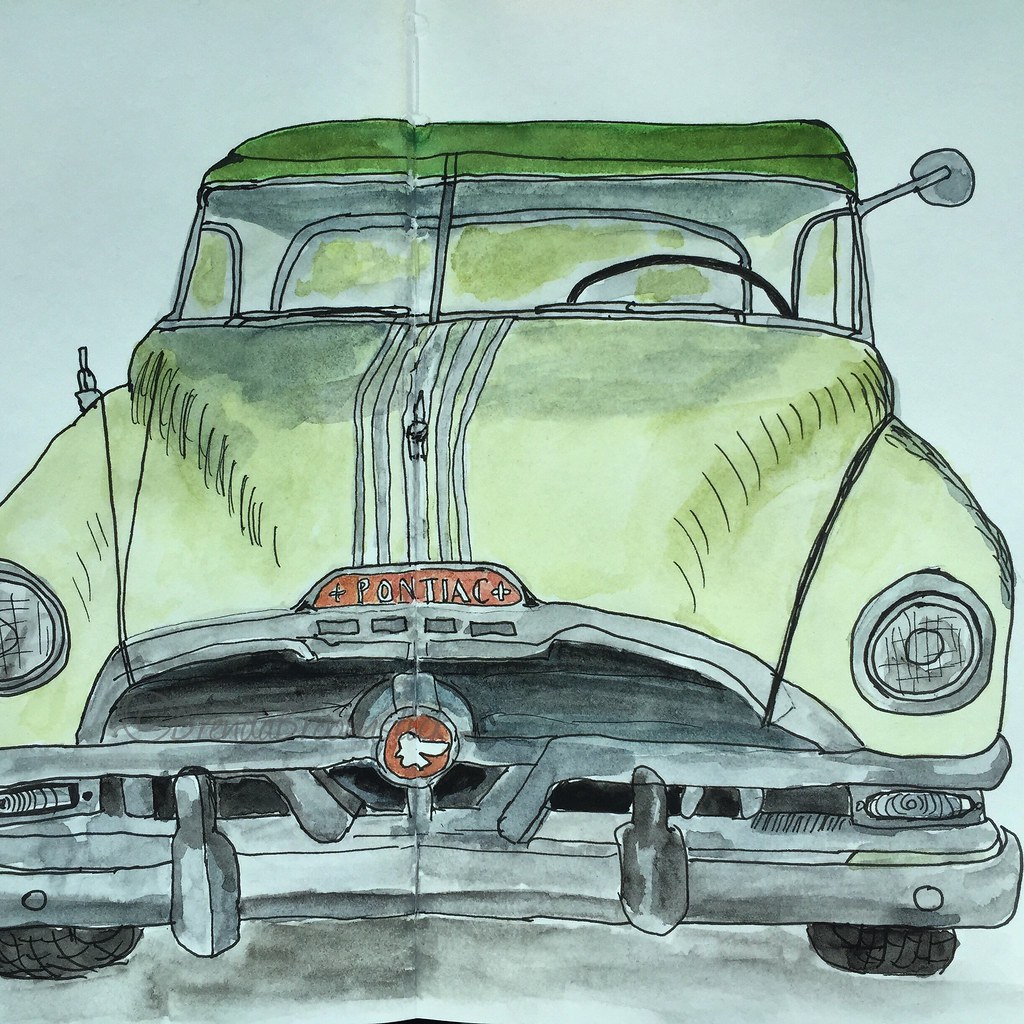This hand-drawn illustration features a front-facing view of an old-fashioned Pontiac car, likely from the 1920s to the 1950s. The car's prominent green bodywork is accented with chrome detailing around the headlights, front bumper, and the single rear-view mirror that diagonally juts out from the right-hand side. The Pontiac logo, set against a red background, is prominently displayed above the simple, heavy, steel-looking grille which consists of four squares. The image highlights the tall, muscular hood and the two-piece windshield, characteristic of older vehicles. The black steering wheel, resembling an arch, can be seen through the windshield on the right-hand side. Beneath the front chrome bumper, the left and right front tires are visible, shaded in various greys and blacks, with tread details peeking out. Notably, the drawing appears to be on a piece of paper that has a crease down the center, suggesting it has been folded.